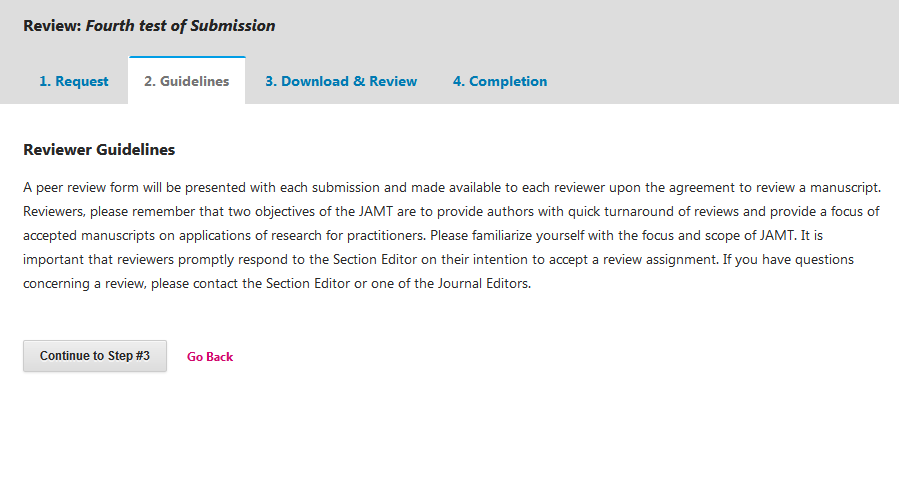This digital image displays the interface of a review submission platform. At the top of the screen, the title "Review Fourth Test of Submission" is prominently displayed. Adjacent to the title is a "Request" button, enhancing user actions. The "Guidelines" tab is highlighted, indicating the current section.

Beneath this, the heading "Reviewer Guidelines" is presented in bold text, drawing attention to its importance. The guidelines inform reviewers that each submission will be paired with a peer review, accessible to each reviewer once they agree to evaluate a manuscript. Instructions emphasize that reviewers must aim for a quick turnaround to assist authors and should prioritize the applicability of research for practitioners, aligning with the focus of the Journal of Applied Management and Technology (JAMT).

Further emphasis is placed on reviewers' responsibility to promptly inform the section editor of their decision to accept a review assignment. Any questions regarding the review process should be directed to the section editor or another journal editor for clarification.

At the bottom of this interface, a gray "Continue to Step Three" button is visible, indicating the next step in the submission process. To the left of this button is a red "Go Back" link, allowing users to navigate to the previous page.